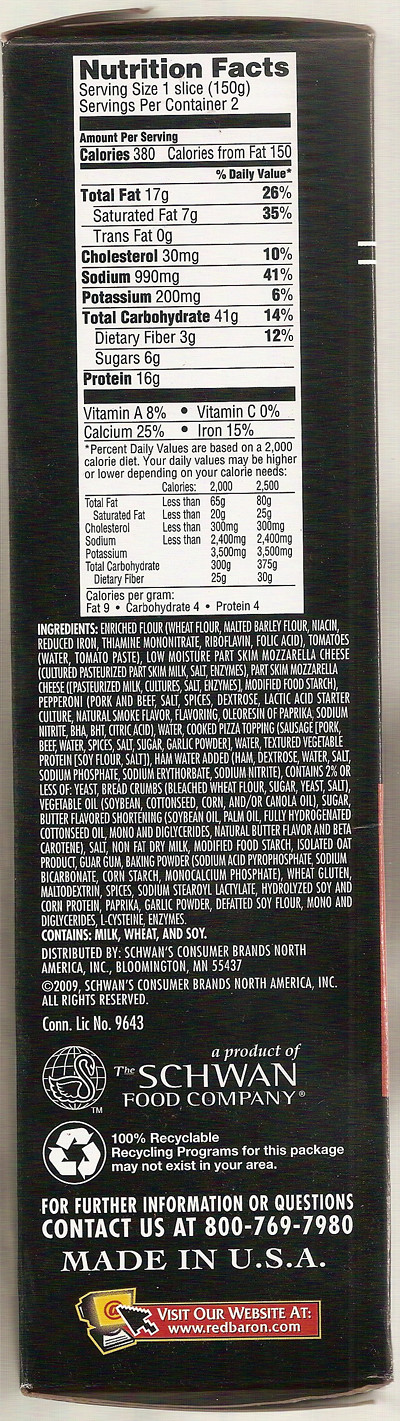This image captures the side of a black cardboard box, likely packaging for a frozen food product such as Red Barron pizza. At the top of the box, there is a white vertically oriented rectangle featuring the heading "Nutrition Facts" in dark letters. Below this, it details the nutritional information, specifying that a serving size is one slice and there are two servings per container. The nutritional breakdown includes: Calories: 380, Total Fat: 17g, Saturated Fat: 7g, Trans Fat: 0g, Cholesterol: 30mg, Sodium: 990mg, Potassium: 200mg, Total Carbohydrate: 41g, Dietary Fiber: 3g, Sugars: 6g, and Protein: 16g. Additionally listed are vitamins and minerals such as Vitamin A, Calcium, Vitamin C, and Iron, with a note that the percent daily values are based on a 2,000 calorie diet and may vary according to individual calorie needs.

Towards the bottom of the box, there is a logo resembling planet Earth with a swan inside, next to the text "A Product of the Schwan Food Company." Adjacent to this is a recycling symbol accompanied by the message "100% recyclable," along with a disclaimer that recycling programs may not exist in all areas. For further inquiries, the packaging provides a contact phone number (1-800-769-7980) and notes that the product is made in the USA. It also includes a website link, www.redbarron.com, indicating this is a Red Barron product, likely containing two slices of frozen pizza.